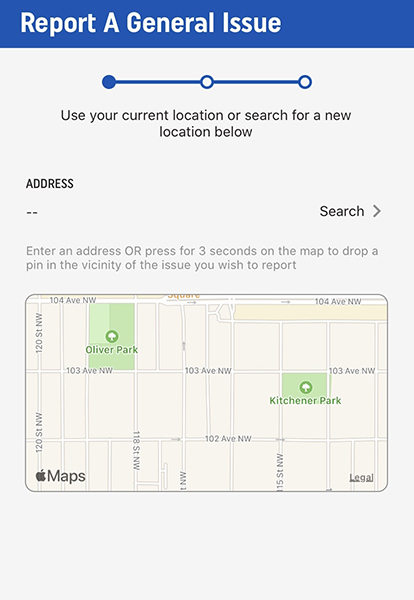The image depicts a tablet screenshot of a website or app interface designed for reporting general issues. The top of the screen features a blue rectangular header with the text "REPORT A GENERAL ISSUE" displayed in white, capitalized letters. Below the header, a linear progress indicator shows three equally spaced dots; the first dot is filled in, while the second and third dots remain empty, suggesting the user is on the first step of a multi-step process.

The interface prompts the user to either use their current location or search for a new location. There's a blank address field accompanied by a search button, allowing users to input an address. Additional instructions advise that users can enter an address or press for three seconds on the map to drop a pin near the issue's location.

The map displayed in the screenshot appears to be Apple Maps, showing a predominantly residential area. Notable landmarks include Oliver Park located towards the top left and Kitchener Park situated towards the middle right of the map. The area is crisscrossed with several streets including 104 Avenue NW, 120 Street NW, 118 Street NW, 103 Avenue, 102 Avenue, and 115 Street. This detailed map view assists users in accurately pinpointing the location of the issue they wish to report.